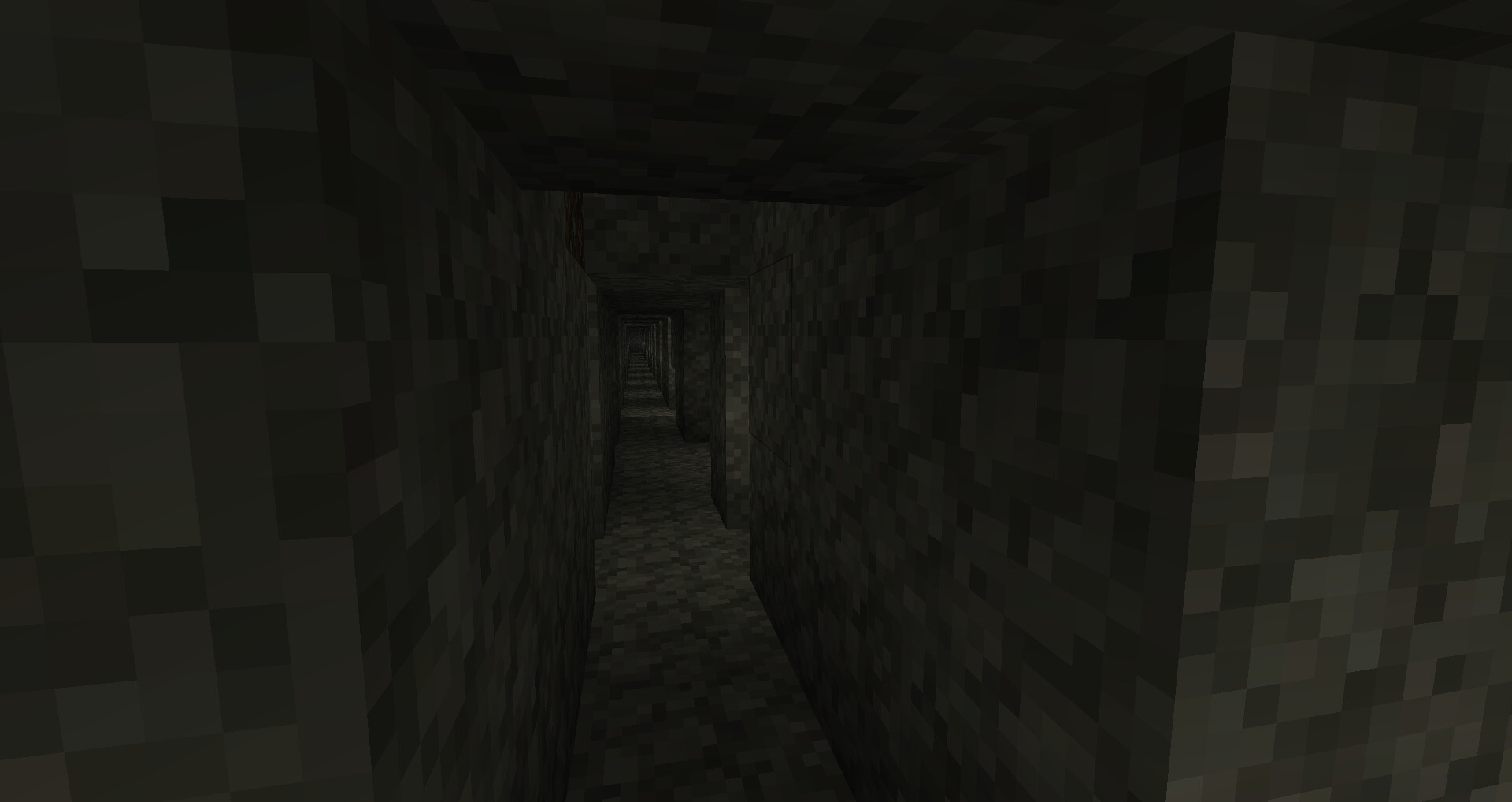A dark-hued, computer-generated image depicting a corridor from a higher vantage point. The scene does not resemble real life but rather evokes a digital, pixelated aesthetic reminiscent of a Minecraft environment. The hallway extends far into the distance, with numerous doorways and openings allowing light to spill into the corridor. The walls are constructed from alternating shades of black and cream-colored squares, creating a textured, mosaic-like pattern. Only two walls are fully visible, indicating that the vantage point is near one of the openings. The corridor appears to stretch significantly, though the exact number of doorways is difficult to ascertain due to the darkness and length of the hallway.